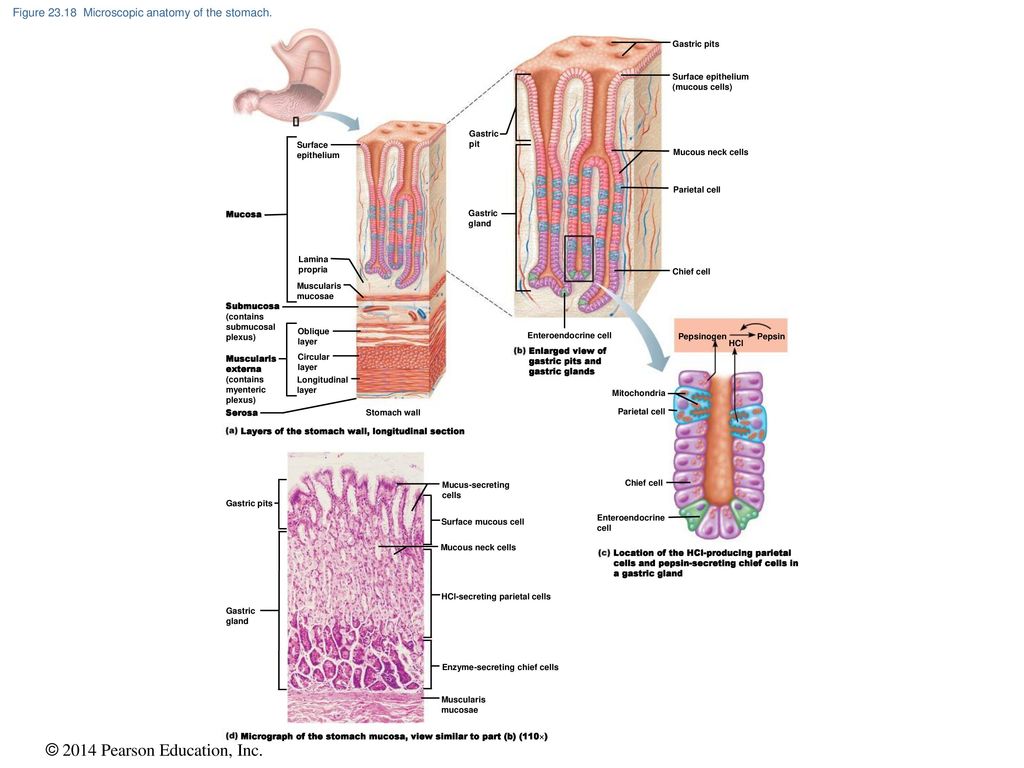The image represents educational content typically found in a science or medical textbook, specifically focusing on the microscopic anatomy of the stomach. Set against a white background, the detailed grayscale diagrams are labeled as Figure 23.18 and illustrate various layers and structures of the stomach wall. These include cross-sections of the stomach showing the surface epithelium, gastric pits, glands, chief cells, and paracellular cells. The image includes a progression marked by arrows between the first and second visuals to show how sections are magnified. There are four distinct cross-sectional diagrams, each meticulously labeled to demonstrate how these cellular components work together to protect the body from infection and disease. The lower left corner of the image bears a 2014 copyright by Pearson Education Incorporated, confirming its authoritative source. The text accompanying the diagrams is small and highly detailed, indicative of its educational purpose.